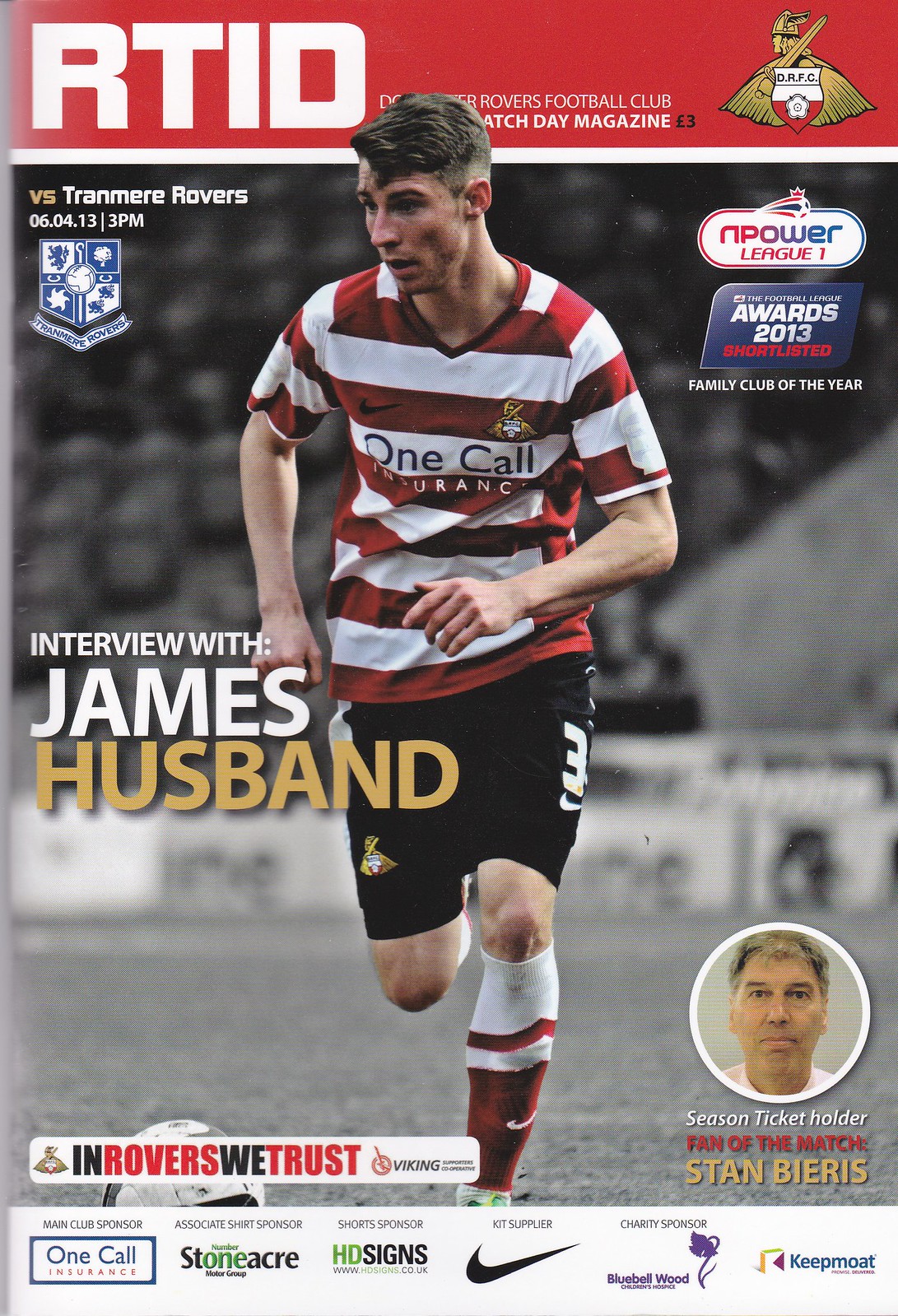The cover of the magazine prominently features a central photograph of a Caucasian soccer player with short brown hair, wearing a red and white horizontally-striped jersey. The jersey bears the logo "One Call Insurance" at the center, with a black Nike swoosh on the left and a gold-and-blue soccer crest on the right. The player is also adorned in black shorts, featuring white stripes, the number three, another white Nike symbol, and knee-high socks that are predominantly white with burgundy accents. 

Above the player, in bold white text against a red background, the title reads "RTID," indicating it is a match day magazine for the Rovers Football Club. To the top right, there is the logo for "Npower League One," accompanied by a smaller dark blue badge that says "Awards 2013 Shortlist" with "Family Club of the Year" written beneath. To the top left, under the RTID header, further text indicates a match against Tranmere Rovers, with the white and blue Tranmere crest adjacent to it.

On the left side of the image, text announces "Interview with James Husband," with "Husband" highlighted in gold. At the bottom right, a circular photograph of a middle-aged man with scraggly gray hair, labeled "Season Ticket Holder Fan of the Match Stan Beers," is featured against a cream-colored backdrop. Next to this image, the text reads "In Rovers We Trust," with "N" and "We" in black, and "Rovers" and "Trust" in red on a white background.

At the very bottom of the cover, logos of various sponsors are lined up, including One Call Insurance, Stone Acre, HD Signs, Nike with its black swoosh, Bluebell Wood with a purple flower, and Keepmoat in blue text. The player's head slightly obscures part of the title, emphasizing his central action in what seems to be a chase for the football on a monochrome stadium background, contrasting with his colorful depiction.